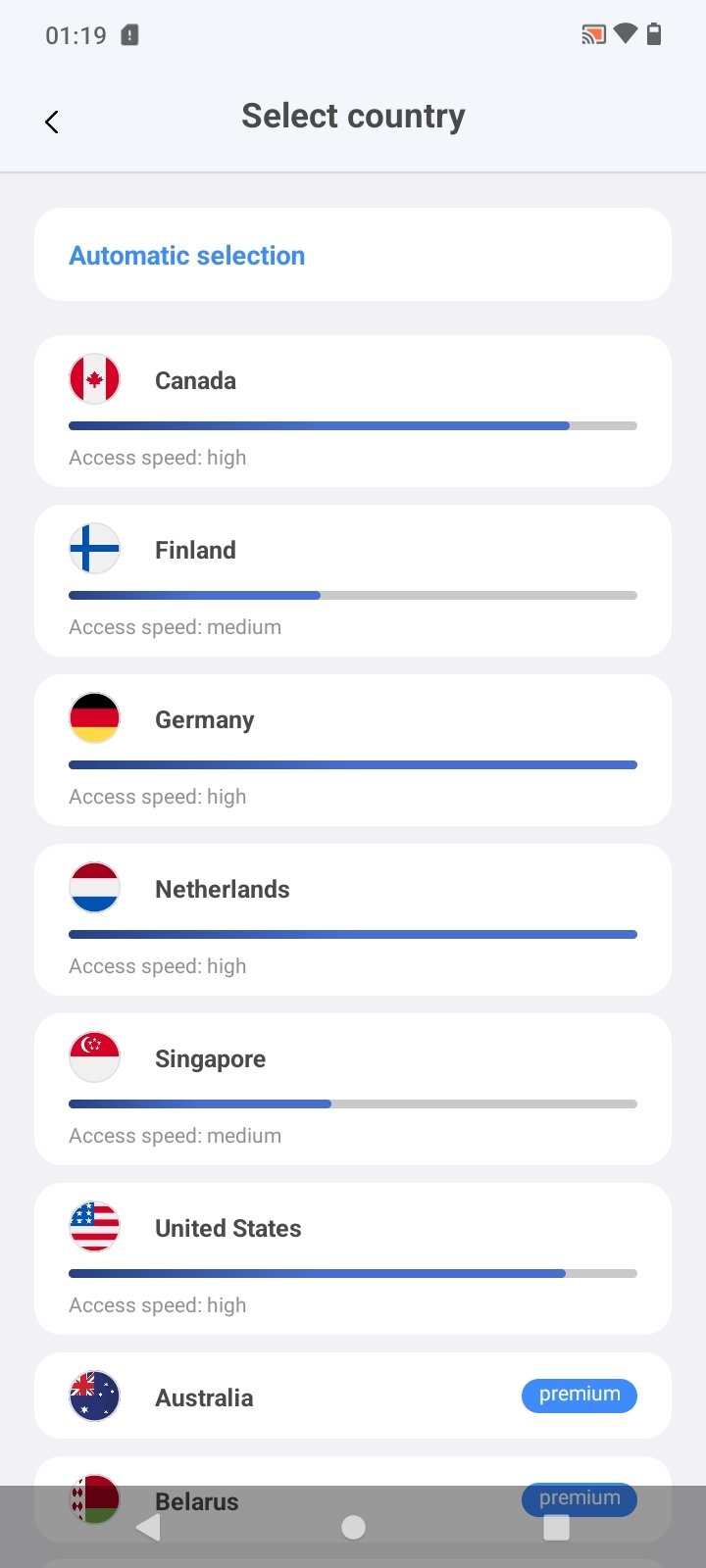**Caption:**

This screenshot captures a mobile phone display. The background is white, with the time "01:19" displayed in the top left corner. To the right of the time, a nearly full battery icon is visible. Below this, a section titled "Select Country" is prominently featured, complete with a list of countries available for selection. Each country's entry includes a flag icon, the country's name, and a corresponding access speed indicator. The options listed are:

1. **Canada**: Flag of Canada, Access Speed: High.
2. **Finland**: Flag of Finland, Access Speed: Medium.
3. **Germany**: Flag of Germany, Access Speed: High.
4. **Netherlands**: Flag of the Netherlands, Access Speed: High.
5. **Singapore**: Flag of Singapore, Access Speed: Medium.
6. **United States**: Flag of the United States, Access Speed: High.
7. **Australia**: Flag of Australia, Access Speed: High, marked with a blue circle labeled "Premium."
8. **Belarus**: Flag of Belarus, Access Speed: Premium, denoted by a blue circle labeled "Premium."

Each entry is succinct and clearly formatted, facilitating quick decision-making for the user.